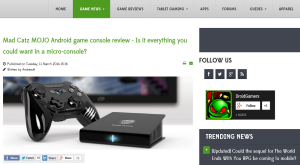**Detailed Caption:**

The image depicts a review webpage for the Mad Catz Mojo Android Game Console. At the top of the page, there is a navigation bar with eight clickable links. The currently selected link is highlighted in green with white text, while the other seven links are in gray with black text, although their labels are difficult to discern. 

Below the navigation bar, the title of the article is prominently displayed as "Mad Catz Mojo Android Game Console Review: Is it everything you could want in a microconsole?" The byline and publication date are just beneath the headline. 

The main image within the article shows the Mad Catz Mojo game console and its controller. The black controller is similar in appearance to a PlayStation controller, although the button layout differs slightly. The console itself is a small, black box resembling an open book turned on its side, featuring a blue light at the front. Both the console and controller rest on a white table. 

In the background, a black TV is mounted on a white wall. While the TV screen is on, the content is not clearly visible, displaying a mix of blue, red, white, and gray hues.

Below the main image, there are social media share links for Facebook, Twitter, Pinterest, and Google. To the side, there is a vertical blue bar labeled "Follow Us," followed by social media icons and the site logo. Further down, a blue box labeled "Trending News" appears, though the stories within are unreadable. A small green square accompanies the white text inside this section.